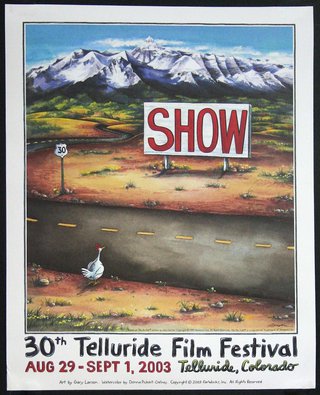This poster advertises the 30th Telluride Film Festival, held from August 29th to September 1st, 2003, in Telluride, Colorado. Created by artist Gary Larson, it features a painterly yet graphic style. At the center of the image, a chicken stands poised to cross a twisty road marked with a Highway 30 sign. The road leads towards a large white roadside billboard with bold red capital letters spelling out "SHOW." Snow-capped mountains and a blue sky frame the background, blending with green and brown fields that evoke the picturesque landscape of the Rockies. The whimsical scene prompts the viewer to ponder, why did the chicken cross the road? Clearly, it’s to get to the SHOW at the Telluride Film Festival. Additional lettering at the bottom of the poster provides festival details and credits the artist, albeit the finer print is difficult to discern.